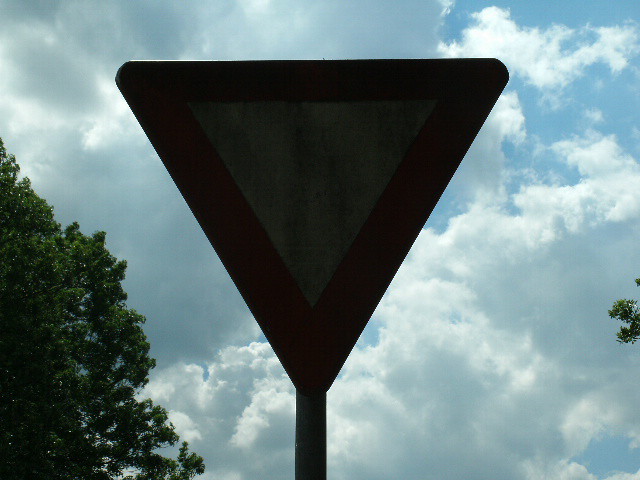The photograph captures a landscape dominated by a cloudy sky, with approximately 80% of it covered by various shades of clouds, ranging from gray to white, hinting at a possible rain. The top right corner of the sky shows some blue patches, while the upper left is dominated by grayer clouds. Nestled in the lower left corner, a lush green tree canopy, likely in full summer foliage, adds a burst of verdant color. The centerpiece of the photo is an old, weathered yield sign, mounted on a metal pole at the bottom center of the image. The sign, an upside-down triangle with a red border and an off-white interior, appears dirty and faded, possibly due to years of exposure. The lighting, seemingly natural and coming from behind, casts a shadow over the sign, reducing its brightness and obscuring any text that might typically indicate "YIELD." The combination of the darkened sign and the cloudy backdrop conveys a somewhat somber, overcast mood.